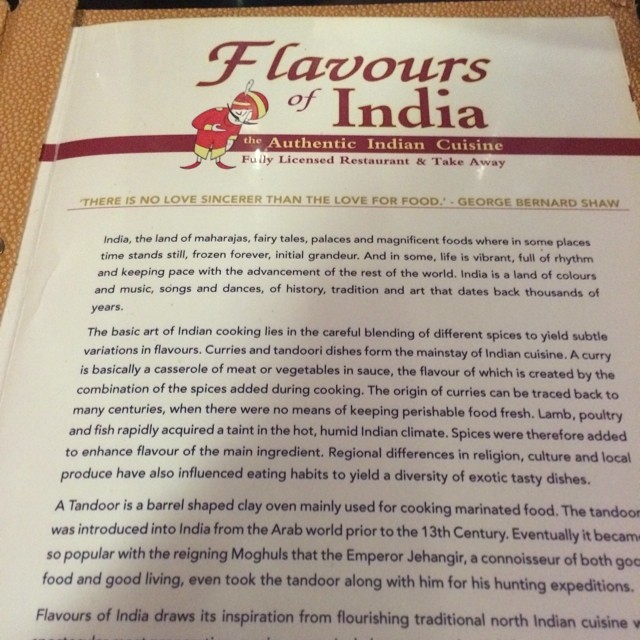This photograph depicts a menu from a restaurant called Flavors of India, placed on a light brown surface. The menu, printed on white paper, has bold red text at the top that reads "Flavors of India." Below, a cartoon character is illustrated flanked by the text, "The Authentic Indian Cuisine, Fully Licensed Restaurant and Takeaway." A notable quote by George Bernard Shaw, "There is no love sincerer than the love for food," is written in green. 

The menu features a detailed introduction to Indian culture and cuisine, composed of several paragraphs in black text. The first paragraph immerses the reader in the rich heritage of India, describing it as a land of maharajas, fairy tales, palaces, music, and dances, where time sometimes stands still or moves vibrantly with modern advancements. 

Further paragraphs delve into the essence of Indian cooking, focusing on the blending of spices to create subtly varied flavors in curries and tandoori dishes. The text explains that curries are casseroles of meat or vegetables in a sauce, with flavors developed through a combination of spices, and how regional differences have contributed to a diverse and exotic culinary tradition. It also details the tandoor, a barrel-shaped clay oven introduced from the Arab world before the 13th century and popularized by the Mughal Emperor Jahangir, known for his love of fine food and living.

This comprehensive description encapsulates the essence of the menu, providing a vivid portrayal of the cultural and culinary treasures highlighted by Flavors of India.